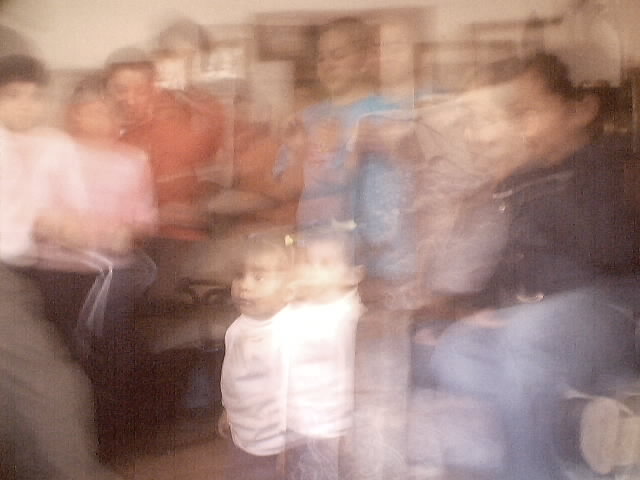In this intensely blurry photograph, a family appears to be gathered, possibly welcoming some visitors. The setting seems to be a cozy living room, though the image’s lack of clarity makes it challenging to discern many details. Central in the scene is a small child, likely around two years old, who appears as a double image due to the blur, making it seem as though there are two overlapping children. On the left side, there is what appears to be a young boy. Next to him, a woman, possibly being embraced by a man whose face is nestled against the top of her head, is present. Following them is a little girl, seemingly around the age of 10 or 11, dressed in a light blue shirt. On the far right, stands another figure, whose gender is indeterminate, dressed in a navy blue shirt and light blue jeans. The background shows various pictures hanging on the walls, though the blur renders their details indiscernible, creating a ghostly effect of duplicates behind the subjects.